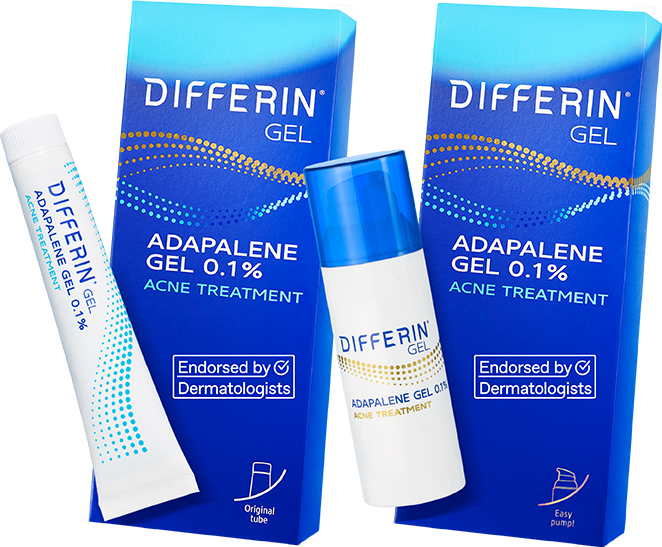The image showcases a series of skincare products designed for acne treatment. The background is white, prominently featuring two distinct packaging types of Differin Gel (Adapalene Gel 0.1% Acne Treatment). On the left side of the image, there is a tilted white tube adorned with blue dot designs, labeled "Adapalene Gel 0.1% Acne Treatment." This tube is complemented by a corresponding blue rectangular box that also bears the Differin Gel branding, complete with blue and gold dot designs arranged in a twirl pattern. The box includes additional details: it states "Endorsed by Dermatologists" with a small check mark and at the bottom right, it specifies "Original Tube."

To the right of this setup, another white container is displayed—this time a pump bottle with a blue cap. The pump bottle features identical branding and labeling: "Differin Gel, Adapalene Gel 0.1% Acne Treatment," and also sports blue dot designs. The accompanying box for the pump bottle is similar to the first, marked by the same dot twirl patterns and branding. However, the box for the pump designates "Easy Pump" at the bottom right, making this the primary distinction between the two available product formats.